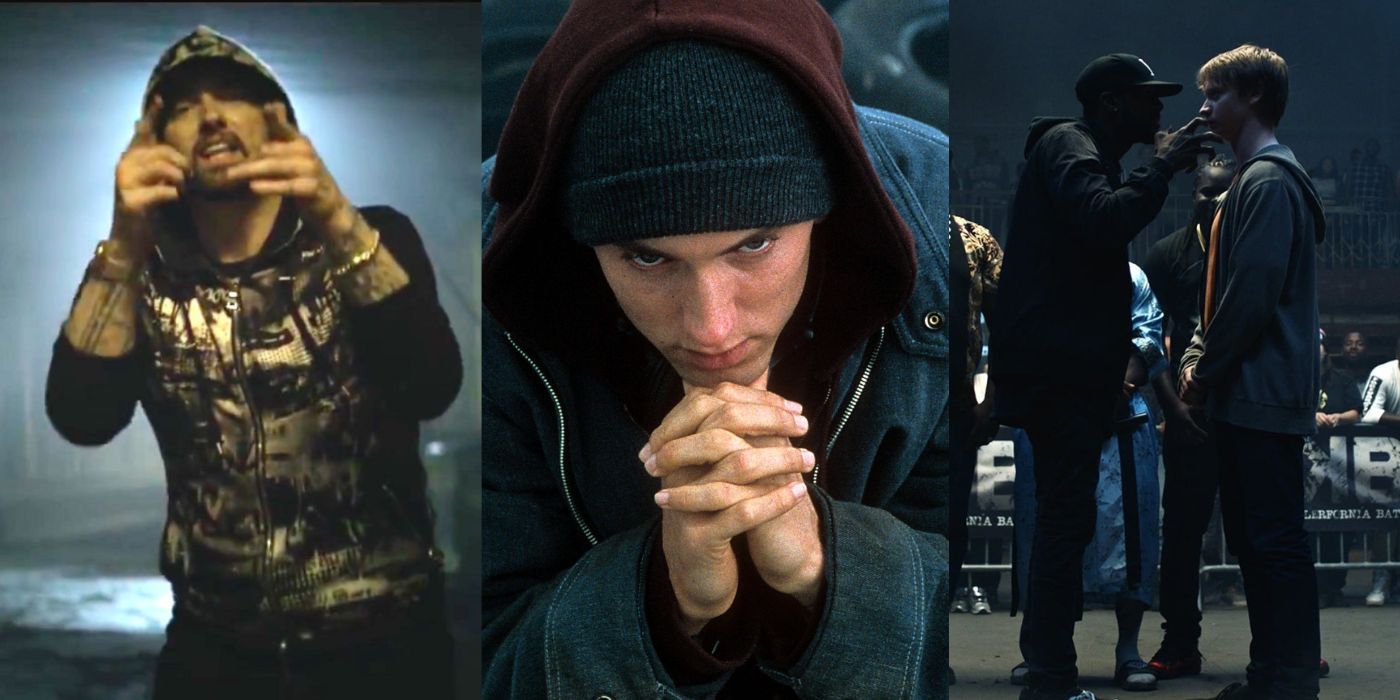The image collage consists of three photographs featuring Eminem, the renowned rapper, and they are quite distinctive in their portrayals. 

In the first image on the left, Eminem is captured in a dynamic and somewhat blurry shot, wearing a shiny black and gold hoodie with the hood drawn up over his head, partially shadowing his face. He is pointing directly at the camera with a finger-gun gesture and appears to be in the midst of speaking or rapping. The background is dark and indistinct, but a bright light encircling his head gives him an almost halo-like aura.

The middle image presents a younger Eminem, reminiscent of his "8 Mile" era. He is clad in a blue jacket layered over a maroon hoodie with a charcoal gray beanie on his head. His hands are clasped together, fingers interlaced, in front of him, and he gazes downward with a serious expression, indicating a pensive or contemplative moment.

The last image on the right is more ambiguous, possibly intended to symbolize a different aspect or representation of Eminem. It depicts a darker-skinned figure, silhouetted and wearing a cap and dark clothing, raising his hand toward another man, likely Caucasian, who stands opposite him and appears to be engaging with or reacting to the gesture. The scene is populated with several other indistinct figures in the background, adding a layer of depth and intrigue.

Overall, the triptych effectively captures Eminem in various guises and moods, from a commanding presence to introspective and then perhaps metaphorical or representational, set against moody and dimly lit backdrops.